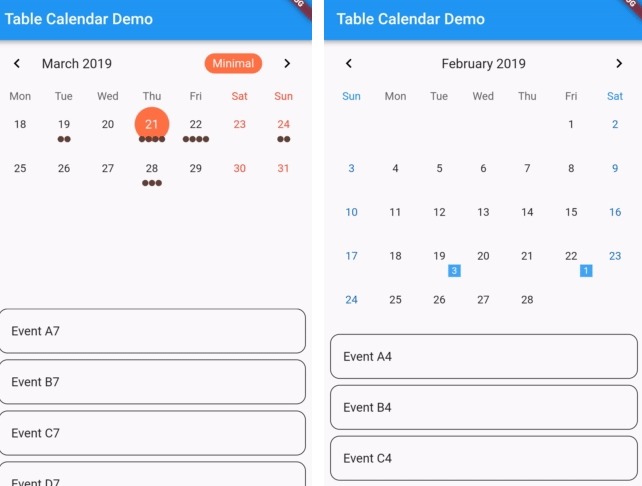This image showcases a side-by-side comparison of two calendar screenshots taken from a cell phone. 

On the left, the calendar displays March 2019, while on the right, it features February of the same year. Both calendar images are titled "Table Calendar Demo" in a blue rectangle at the top. In the upper right corner of each blue rectangle, the tip of a red pencil, near its eraser, is visible.

Examining the March 2019 calendar on the left, noticeable details include a couple of areas marked with black dots and a prominent orange circle around the 21st, along with the word "minimal" appearing in the calendar grid. At the bottom of this calendar, the text reads “Event A 7, Event B 7, Event C 7, and Event D 7.”

The February calendar on the right highlights some dates with blue numbers. Unlike the March calendar, its event listings at the bottom are simpler, stating only “Event A 4, Event B 4, and Event C 4.”

These differences between the two months are clearly depicted, emphasizing the variation in events and visual markers between February and March 2019.